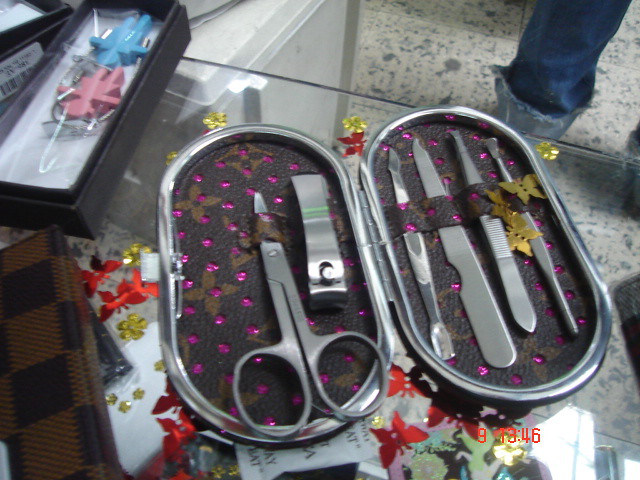This detailed, color photograph captures an assortment of stainless steel manicure and pedicure tools stylishly arranged inside a luxurious, oval-shaped toiletry kit. The kit, likely designed with a nod to high fashion, features a brown, hole-punched lining adorned with the iconic Louis Vuitton logo. Nestled within the kit are a toenail clipper, two pairs of tweezers, a nail file, and manicure scissors, each held in place by designated loops and slots. The interior is accentuated with pink rhinestones, adding a touch of glamour. The kit is situated on a glass countertop, further evidenced by the reflective surface, and nearby, other grooming tools and decorative cases are scattered. In the background, a white cabinet, tiled flooring, and a glimpse of denim-clad legs suggest the setting is a well-appointed, serene salon. Additional decor, including red and gold stickers with the numbers 91346, can be seen along the top area of the table, contributing to the vibrant yet refined atmosphere.